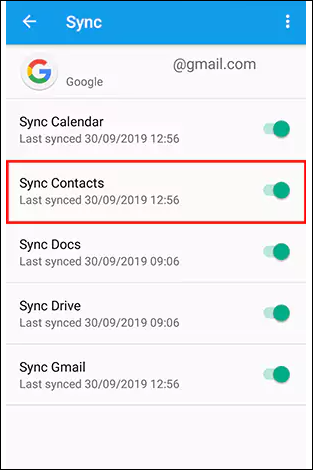The image is a detailed screenshot from the information section of a website, displaying various synchronization options for Google services. Located at the top-left corner, the word "Sync" is prominently featured. Below this, the recognizable Google icon is displayed alongside the word "Google." Adjacent to this, on the right side, an email address ending in "@gmail.com" is visible.

Directly beneath the email address, there are several synchronization options listed: "Sync Calendar," "Sync Contacts," "Sync Docs," "Sync Drive," and "Sync Gmail." Among these options, "Sync Contacts" is distinctly highlighted with a red box encircling it, drawing attention to this specific option. Notably, all the synchronization options were last synced on the same date: September 30th, 2019. This provides a snapshot of the status and options available for synchronizing various Google services.